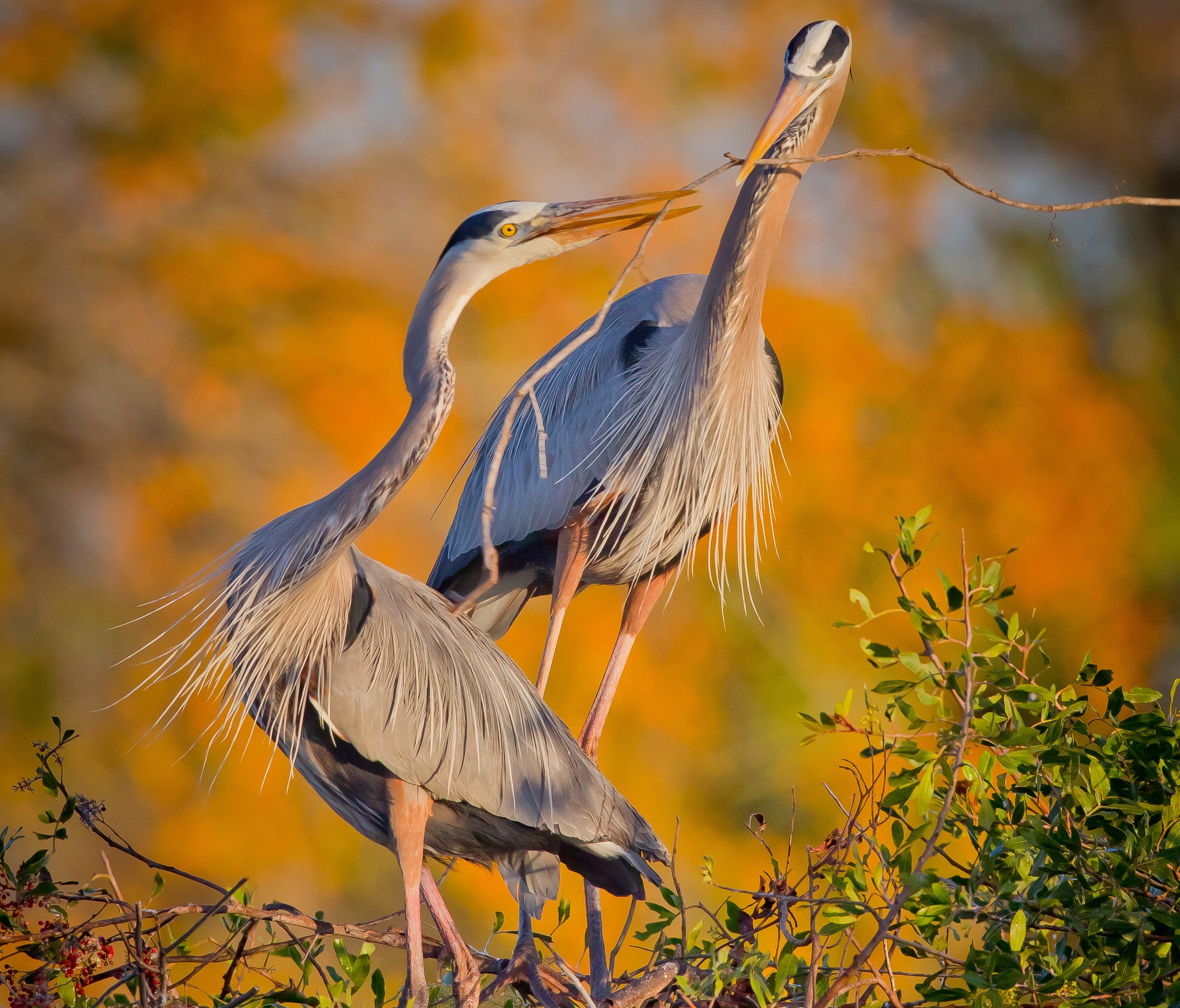In this photograph, two large birds with striking features stand amidst a lush, green landscape. Their long, orangish-pink legs support their gray bodies, which are adorned with fringes of feathers around the neck area that resemble flowing hair. Their slender necks stretch upward, leading to heads that are predominantly white, accented by a distinct black stripe from the eye to the back of the head. Their long beaks are a noticeable orange.

One bird faces the camera directly, while the other is in profile, glancing back. They seem to be tussling over a stick, with one bird gripping it in its beak while the other attempts to take it away. Below them, the ground is scattered with sticks, green leaves, and vibrant red berries. The background is a blur of autumnal orange, with hints of green and blue, highlighting the birds as the focal point of the image.